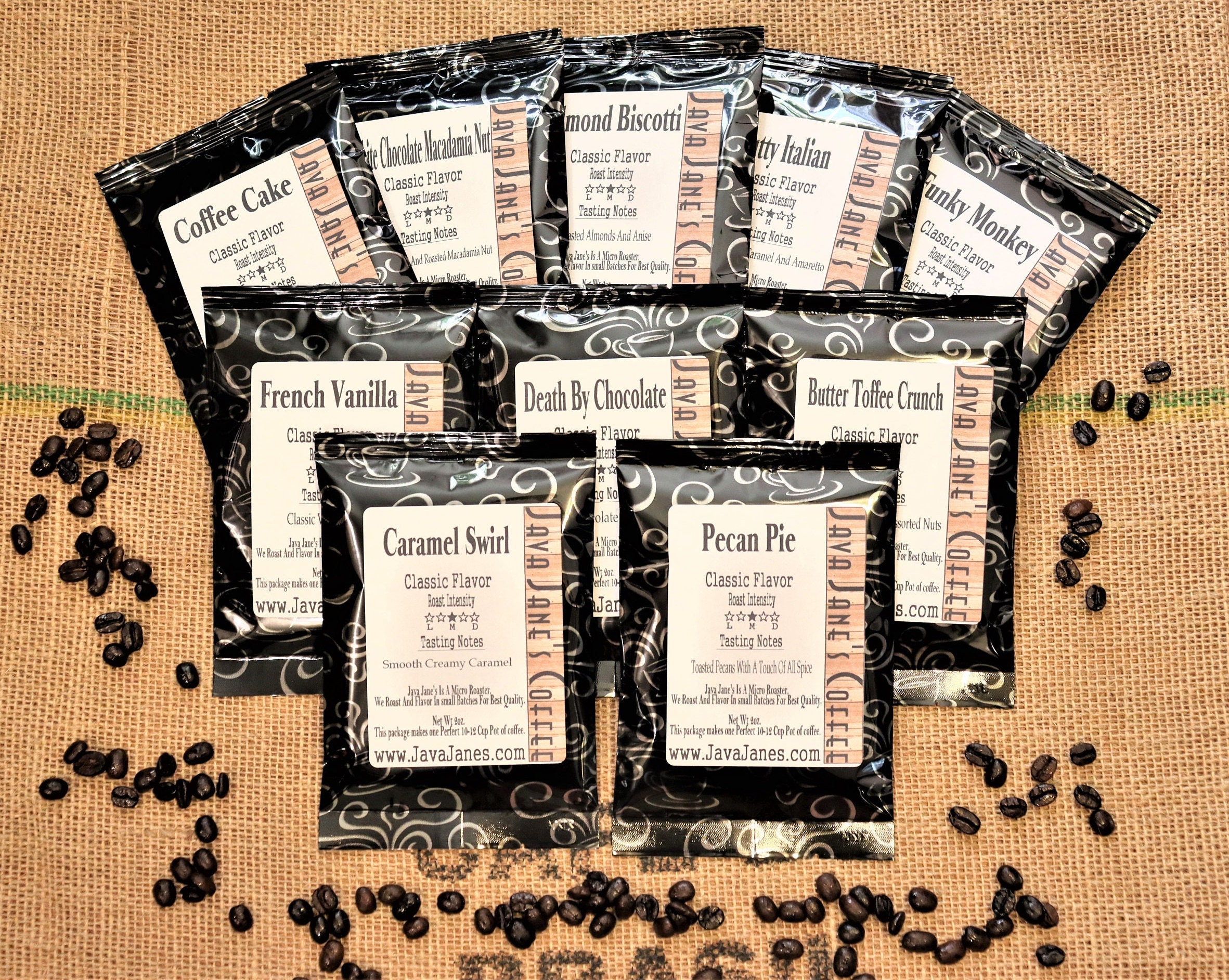The image depicts an assortment of Java Jane's Coffee packages arranged in neat rows against a burlap background, distinguished by a green stripe running horizontally about one-third from the top. The top row features five packages, the middle row has three, and the front row includes two packages, all slightly overlapping. Scattered dark brown coffee beans add a rich texture beneath the green stripe on the left and spread upwards on the right, nestled behind the bags. Each package, crafted in dark brown with white curlicue designs, features a prominent white label adorned with dark brown lettering and a light brown vertical stripe on the right. The visible flavors include Coffee Cake, Almond Biscotti, Funky Monkey, French Vanilla, Death by Chocolate, Butter Toffee Crunch, Caramel Swirl, and Pecan Pie, resembling dessert treats in both name and packaging.